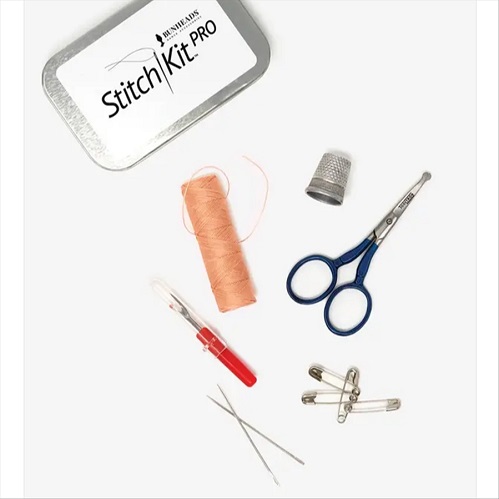This image showcases the contents of the Stitch Kit Pro by Bunheads, neatly arranged on a white table. The top left of the image features a brushed metal tin adorned with a white sticker depicting the silhouette of a woman with a bun hairstyle and the text "Stitch Kit Pro" and "Bunheads." Next to the tin, there's a spool of salmon-colored thread and a silver metal thimble. On the right side, a pair of scissors with a blue handle sits prominently. Below the scissors is a cluster of four safety pins, organized with three clipped to one for neatness. Toward the bottom, a red-handled seam ripper is visible alongside a pair of crossed sewing needles. The objects are scattered but distinctly visible, presenting a detailed view of the kit's components, enhanced by the colors silver, white, off-white, black, peach, blue, and red. The arrangement suggests a display setup, possibly aimed at showcasing the kit's contents for potential buyers.